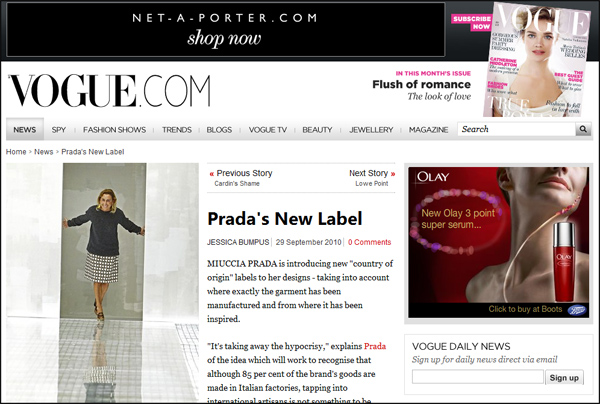This screenshot captures the Vogue.com website, showcasing a sophisticated layout and various elements aimed at engaging the reader. At the very top, there's a sleek advertisement for Net-A-Porter.com, featuring a black background with elegant white text that reads "Net-A-Porter.com" accompanied by the phrase "Shop Now" in delicate cursive.

In the upper right-hand corner, an enticing subscription promotion is displayed. It includes an image of a Vogue magazine cover set against a vibrant pink background with the words "Subscribe Now" in bold white text. The featured cover depicts a light-skinned Caucasian woman adorned in what appears to be an ethereal wedding dress.

The majority of the website features a clean, white background with sharp, black text. Prominently displayed below the ad is the site’s title, "Vogue.com". Adjacent to the magazine cover, a brief description is provided, stating, "In this month's issue: A flush of romance; the look of love."

A navigation menu with a subtle gray background sits below the site title, offering links to various sections such as News, Spy, Fashion Shows, Trends, Blogs, Vogue TV, Beauty, Jewelry, and Magazine. Also present is a search bar for easy access to specific content.

The main body of the webpage includes a striking photograph on the left-hand side, depicting a woman walking through grand, ornate doors. Below this image, a headline announces an article titled "Prada's New Label." Adjacent to this, an advertisement for an Olay product captures attention, seamlessly integrated into the website's stylish and modern design.